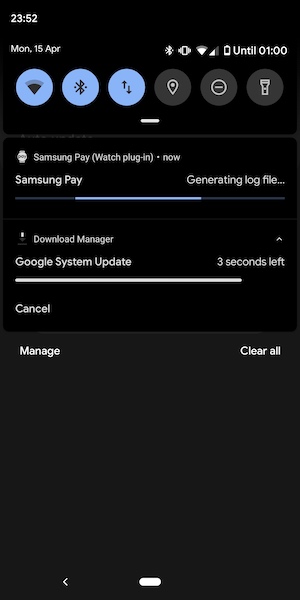This image captures a smartphone screen showing the user's notifications and status bar interface. At the top, there's a status bar displaying several circular icons indicative of active settings, including Wi-Fi, Bluetooth, and a data transfer icon, all highlighted in a bluish periwinkle color, followed by grayed-out icons representing other features such as a pin, mute, and flashlight.

Below the status bar, a notification segment reveals various system updates and information. The first notification is related to Samsung Pay, accompanied by a message indicating "generating log file..." horizontally divided by a bluish periwinkle line.

Further down, there is a download manager notification for a Google system update, specifying "Three seconds left" to completion. Underneath this progress bar, options to "Cancel" on the left and "Manage" on the right are provided in smaller fonts. 

Overall, the screen gives insight into ongoing actions, such as software updates and system logs, amidst an interface interspersed with soft blue and gray thematic elements.